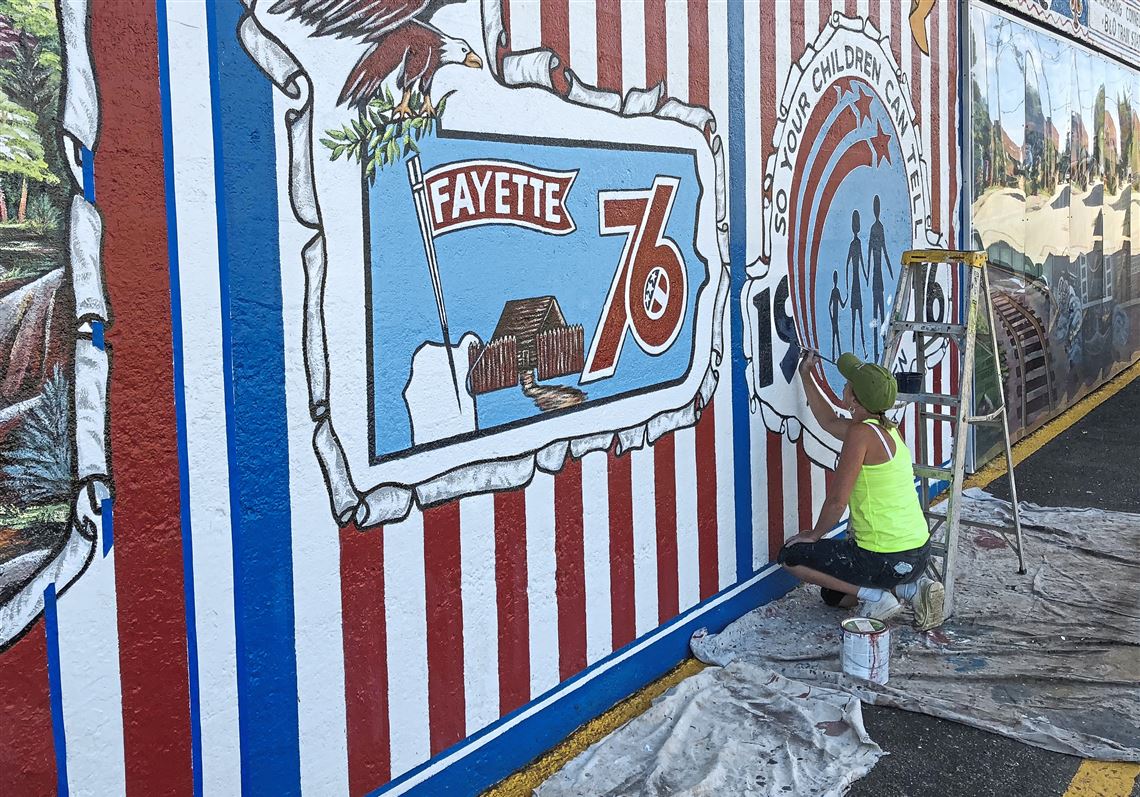In the center-right of the image, a woman is crouched down, hand-painting an elaborate mural. She is wearing a fluorescent green tank top, black shorts, white socks, sneakers, and an army green ball cap. The woman has a paintbrush in hand and a can of paint nearby. Drip cloths, dirty with paint and darker discoloration, are spread on the asphalt in front of her. 

The mural features elements of the American flag, including red and white stripes and blue stripes. In the upper center, a flag on a pole bears the inscription "Fayette 76," with a wood fort depicted underneath. To the right of this scene is another painted element with the phrase "so your children can tell," partially obscured by the woman's position. An eagle perched on the corner of what appears to be the outline of a state, possibly Arkansas, further enhances the mural's complexity. The entire artwork is a rich tapestry of patriotic symbols and historical references.